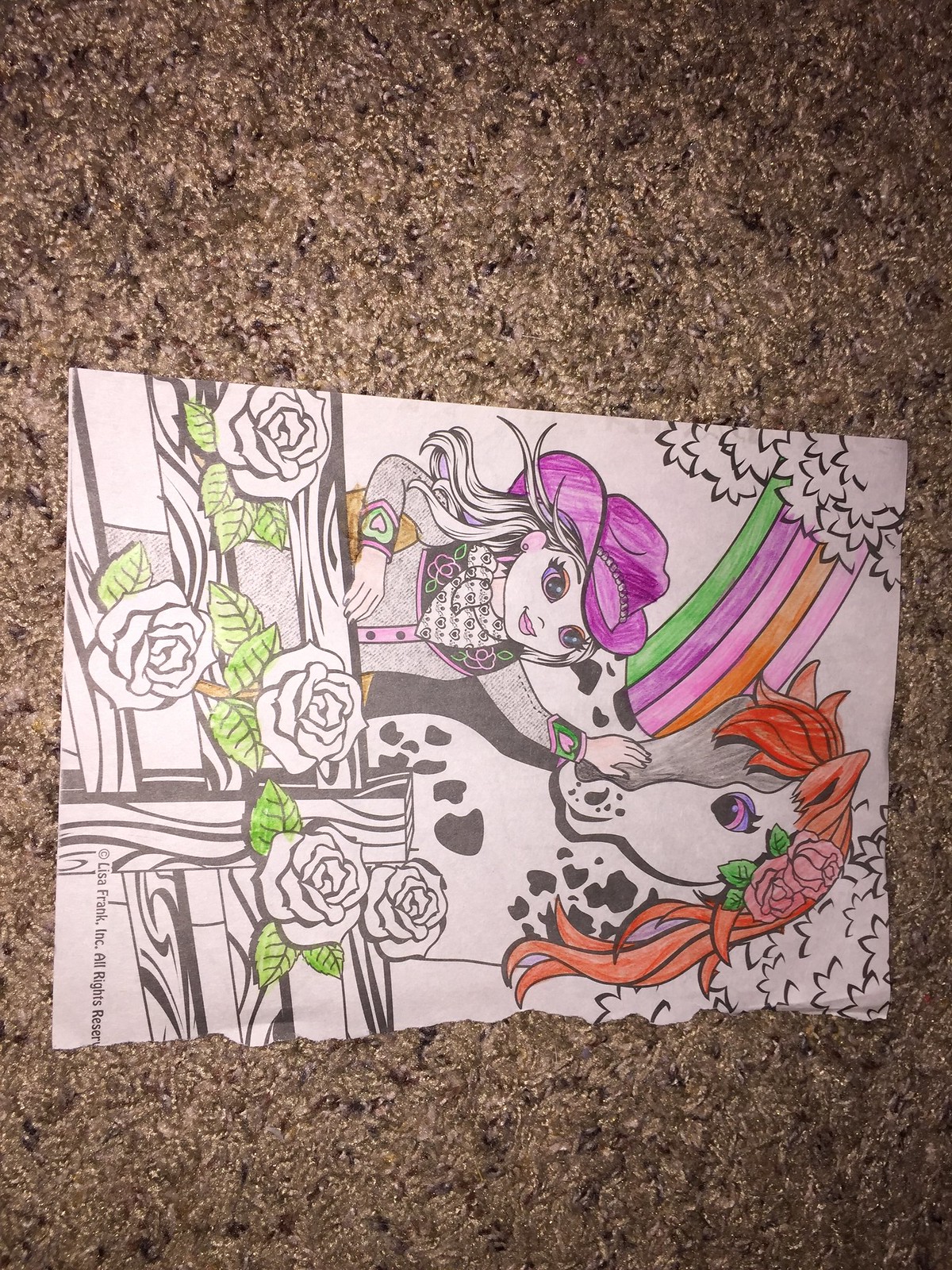This photograph captures an illustration drawn on a piece of white computer paper that lies on a thick, brown, textured carpet resembling the appearance of wild rice. The image is oriented sideways, with the top pointing to the right. The illustration features a girl dressed in a purple cowgirl outfit complete with a hat, gently patting the head of a pony. The pony has striking purple eyes, a long orangish mane adorned with pink roses. A vibrant rainbow, consisting of green, purple, pink, and orange hues, arches behind them. The illustration appears to be a page from a coloring book, characterized by cutesy, large-eyed figures reminiscent of Bratz dolls. Additionally, there is a large fence in the background decorated with uncolored roses, while some green leaves have already been filled in by the artist, showing partial progress in the coloring process.